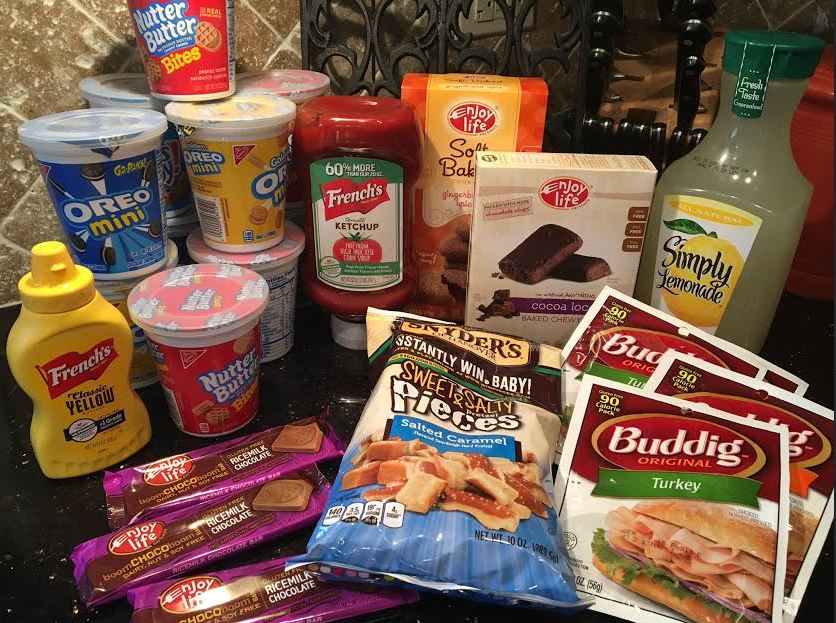The image features an array of groceries meticulously arranged next to each other, likely for organizational or visual impact. Starting from the top left, there are several small canisters of various cookies. The blue canisters are labeled "Oreo Mini," while the red ones are marked "Nutter Butter," and the yellow canisters are identified as "Graham Oreos." 

On the left-hand side of the image, a French's Classic Yellow Mustard bottle stands prominently. In the center, there are packages of Kerschneider's Sweet and Salty Pretzel Pieces. Moving to the bottom right, you can see a package of Butterball Original Turkey and a bottle of Simply Lemonade.

These items create a colorful and varied display, highlighting popular snack and condiment options.